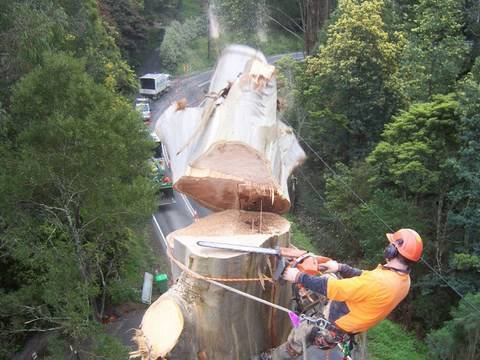This aerial photograph captures a dramatic scene of a tree surgeon, clad in a yellow long-sleeve jacket and red helmet, perched at the top of a tall, branchless tree trunk, approximately 50 to 60 feet above the ground. Supported by a harness and ropes akin to rock climbing gear, the worker is captured in the act of sawing off the top three feet of the tree with a chainsaw, the severed portion caught mid-fall as it tilts backward from the cut. His surroundings include a curving two-lane highway directly below, with several vehicles—a white truck, a small white car, and a gray truck—traversing the road. Flanking either side of the image are dense areas of green forestry, with power lines running parallel to the highway. The scene powerfully conveys both the height and the precision required for such a task.